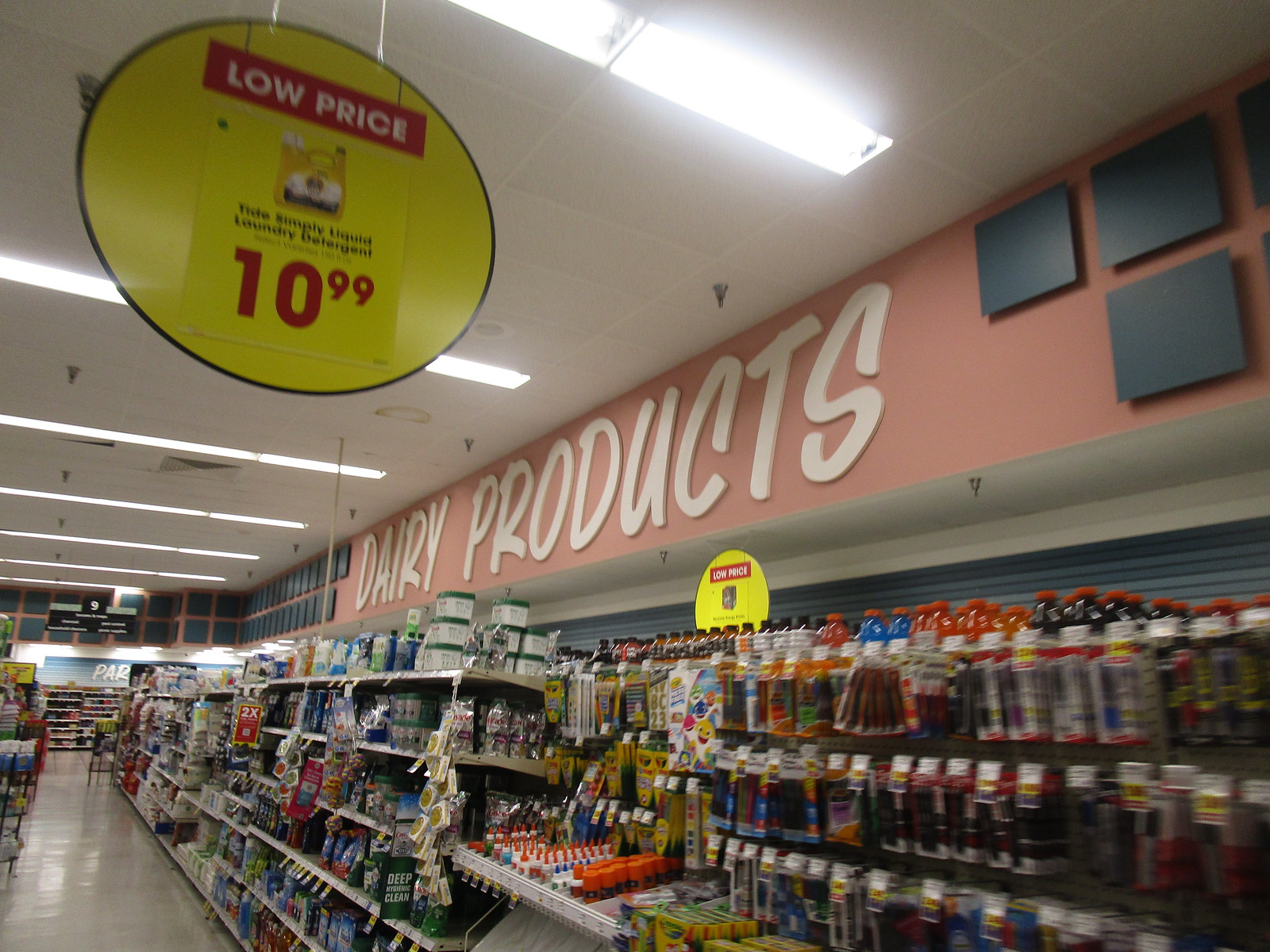This photograph showcases the interior of a grocery store, capturing a vivid, crisp, and clear image. Prominently hanging from the ceiling on the left side of the image is a colorful sign in yellow, red, and white, advertising "Low Price, Tide Simply Liquid Laundry Detergent, $10.99." The store is illuminated by fluorescent lights affixed to a white ceiling. 

A section of the wall, painted in a salmon hue and adorned with white lettering, reads "Dairy Products," accompanied by black square accents. Interestingly, despite the signage, the area below does not contain dairy products. Instead, it is stocked with various bottles of what appears to be Gatorade, each featuring an orange lid and a spectrum of liquid colors including black, orange, and blue.

Further in the background, the image reveals a school supply section. This area is neatly organized, displaying an assortment of pens, boxes of Crayola crayons, and bottles of glue. Nearby, there are also shelves stocked with dishwasher pods and other miscellaneous items, reflecting the diversity of products available in the store. The overall sharpness and detail in the photograph provide a clear and comprehensive view of the store's interior.